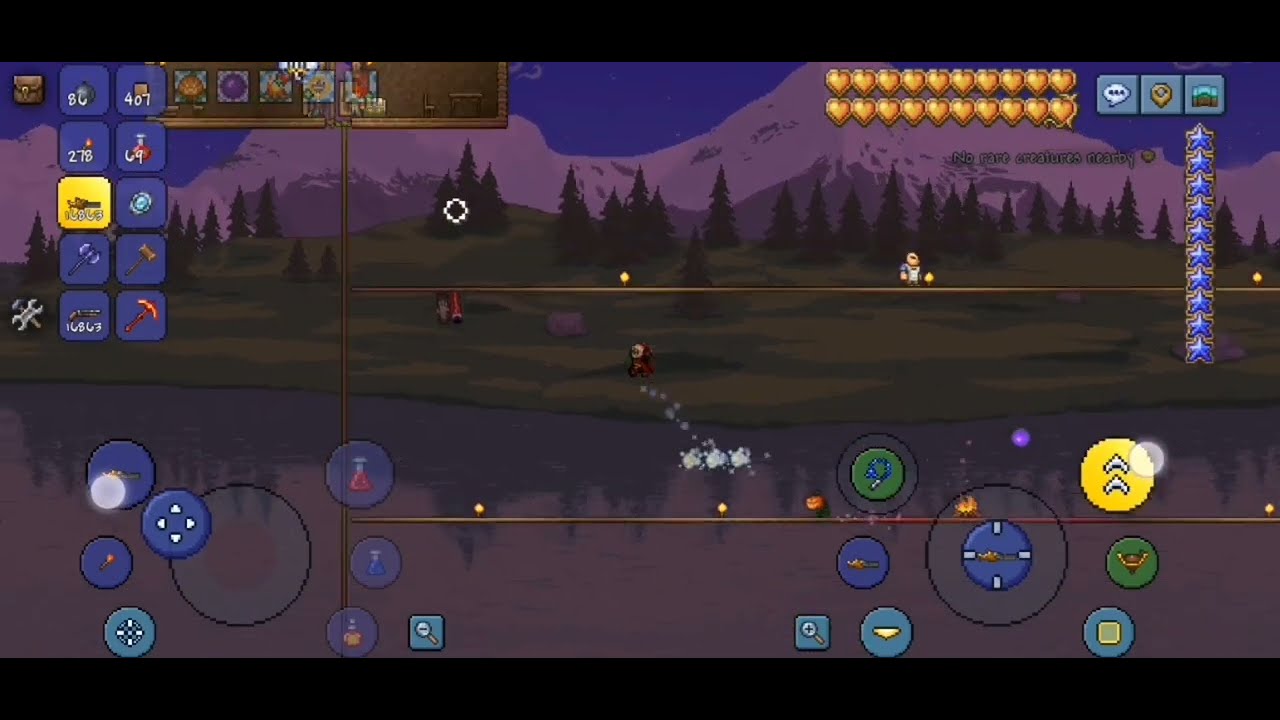The image is a detailed screenshot of a side-scrolling video game, shown in third-person perspective. The scene is set under a starry night sky and features a diverse landscape. At the bottom of the image, there is a lake reflecting portions of the environment. Above the lake, a grassy field with a hilly surface stretches into the distance, where pine trees and snowy mountains can be seen.

The game interface is loaded with graphical elements around the edges. In the upper left corner, there's a character’s inventory displaying items like a hammer, potions, money, bombs, and a gun. Right below this, in the bottom left corner, there are control icons including arrow keys for movement, a map, and a magnifying glass for zooming in.

Moving to the upper right corner, there are two rows of yellow hearts indicating health, alongside blue boxes and a row of blue stars. Additionally, there's a speech bubble, a map, and a vertical line of stars. The bottom right corner features more icons for movement, such as a lamp, arrows, and a compass.

In the central gameplay area, a tiny character is seen walking on the banks of the lake in a forested region with mountains in the background. Nearby, green circles contain icons like a beaker, a magnifying glass, a man, and a downward-pointing arrow. The left side of the screen shows blue circles with various symbols, including arrows and dots, and two rows of blue boxes with numbers, one of which is yellow, sitting above a brown box with unclear icons.

Overall, the screenshot captures a vibrant and complex gaming interface amidst a picturesque natural setting.